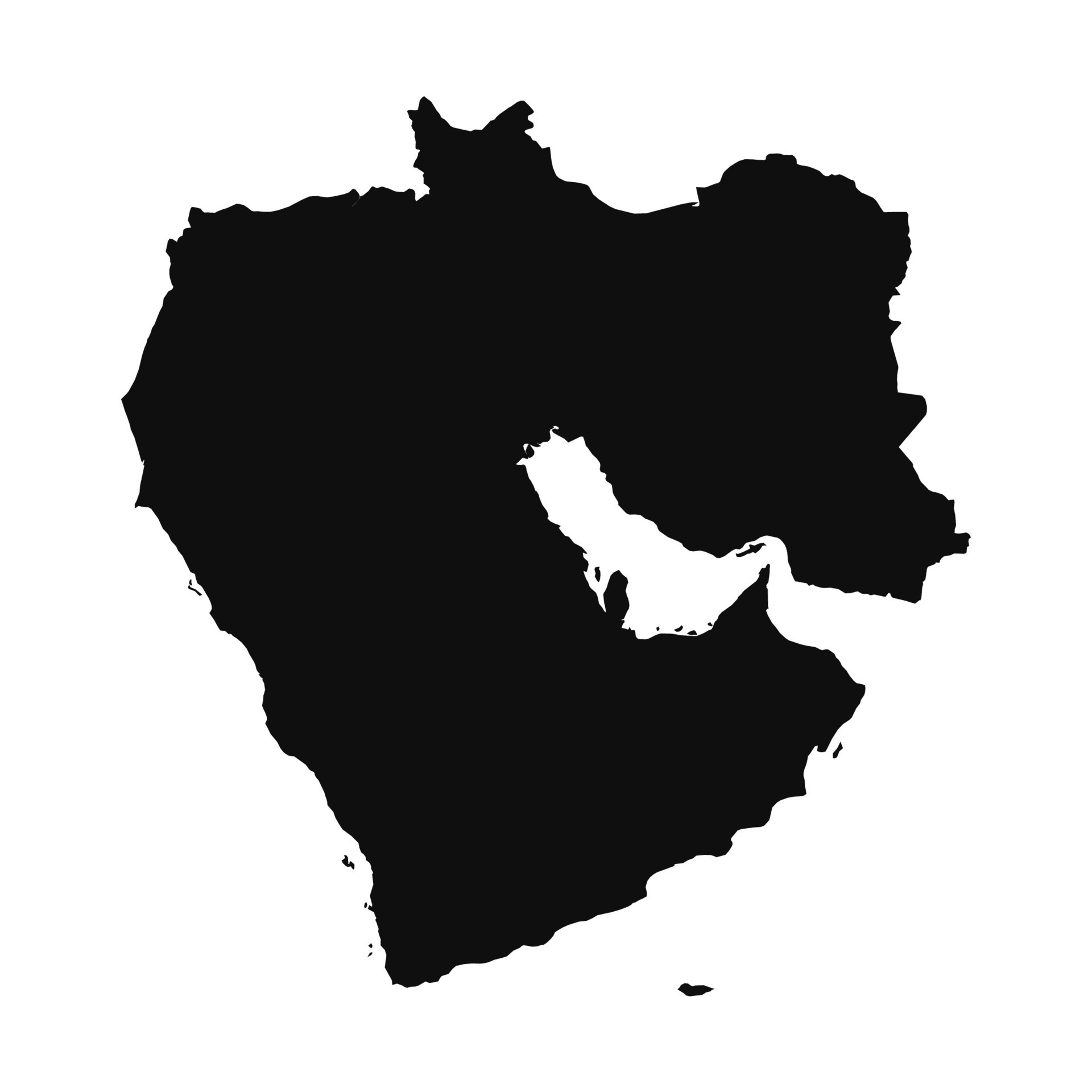This is a simple yet striking black and white abstract silhouette of the Middle East. The entire landmass is colored in black, with surrounding areas, including waterways and borders, left in white, creating a stark contrast. The map omits any detailed separation between countries, leaving regions such as Iran, Iraq, and Saudi Arabia as a singular black area against the white background. The edges of the continents are cleanly profiled, although there appear to be scattered black dots, which may be artistic touches rather than geographical features. The image contains no text or other markings, adding to its minimalist, almost ink-blot-like aesthetic.